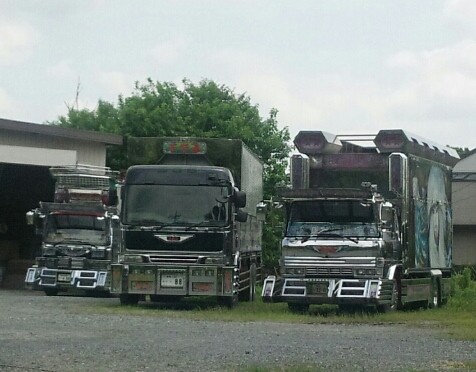This outdoor daytime photograph depicts three distinct large trucks parked side by side on a grassy area, with gravel patches in the foreground and a garage building to the left. The sky is slightly overcast, showcasing light blue with some fluffy white clouds. In the background, a fully bloomed green tree adds to the serene ambiance. 

The truck on the left is the smallest, notable for its intricate chrome grill and bumper, and appears somewhat similar to a heavily modified camper. It sports a red color with an unusual metal structure atop its box section, giving it a rugged, almost "Mad Max" aesthetic.

The middle truck is black, larger than the left, with a sleek, shiny black window. This truck, similar in size to the one on the right, also features ornate chrome elements and looks more like a typical European tractor-trailer rather than a North American one.

The truck on the right is purple and garners attention with a mural-like design on its side. The intricately detailed chrome bumper and grill enhance its imposing presence. This truck is slightly angled, providing a three-quarter view of its decorated side. 

In the background to the left, the garage has a beige structure with a flat brown roof and an open door. Patches of grass sprout through the gravel driveway, blending industrial ruggedness with natural elements. No text or branding is visible on the trucks, signifying their standout uniqueness and possibly customized nature.